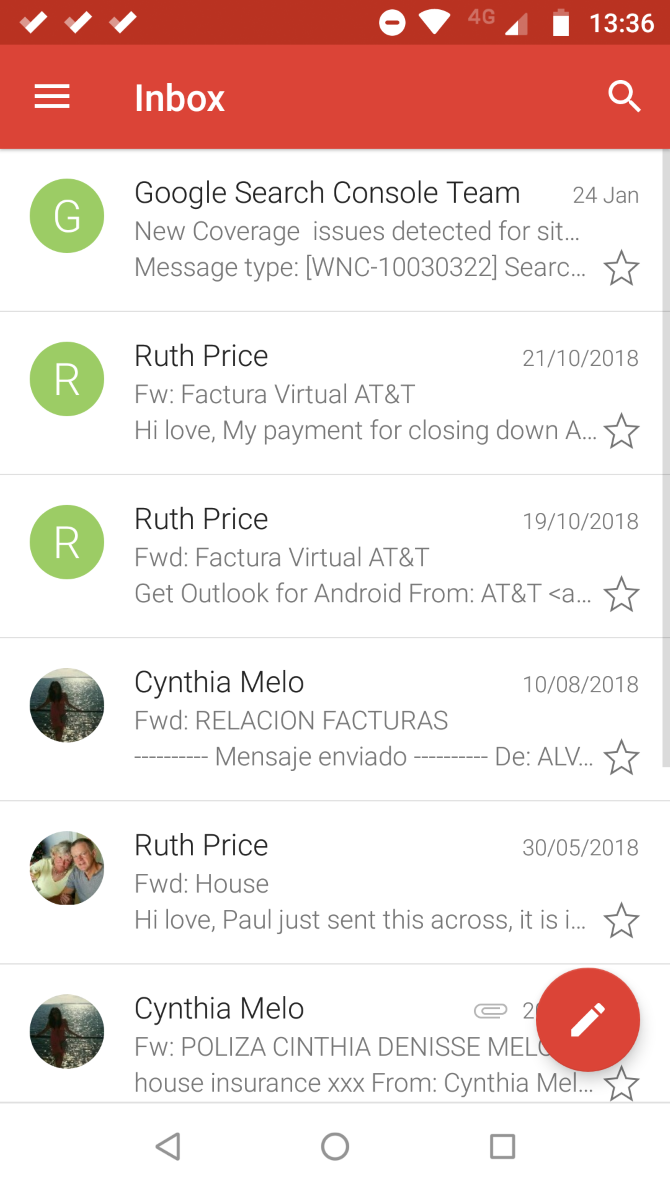The screenshot displays a vertically oriented cell phone screen. At the top, there's a red bar containing various symbols: check marks in the upper left corner, and the time, battery indicator, and Wi-Fi symbol in the upper right corner. Below the red bar, the interface showcases three horizontal white lines forming a square icon on the upper left, labeled "Inbox" in white text to the right of it. Additionally, there is a white magnifying glass icon on the right side, indicating a search function.

The main portion of the screen shows an email inbox against a white background with black text, segregated by horizontal lines. The first email is from "Google Search Console Team," with the subject line reading "New coverage issues detected for sit..." followed by some message identifiers. Each email has an associated colored circle with an initial: the first email has a green circle with a 'G'.

The second email, identified by a green circle with an 'R', is from "Ruth Price" with the subject "Forward Factura Virtual AT&T." The preview reads, "Hi, love. My payment for closing down a..." The third email, again from "Ruth Price" as indicated by the green 'R' circle, shares a similar subject and reads, "Get Outlook for Android from AT&T at..."

In total, there are six messages visible on the screen. At the bottom right, a red circular icon with a white pencil inside symbolizes the compose message function.